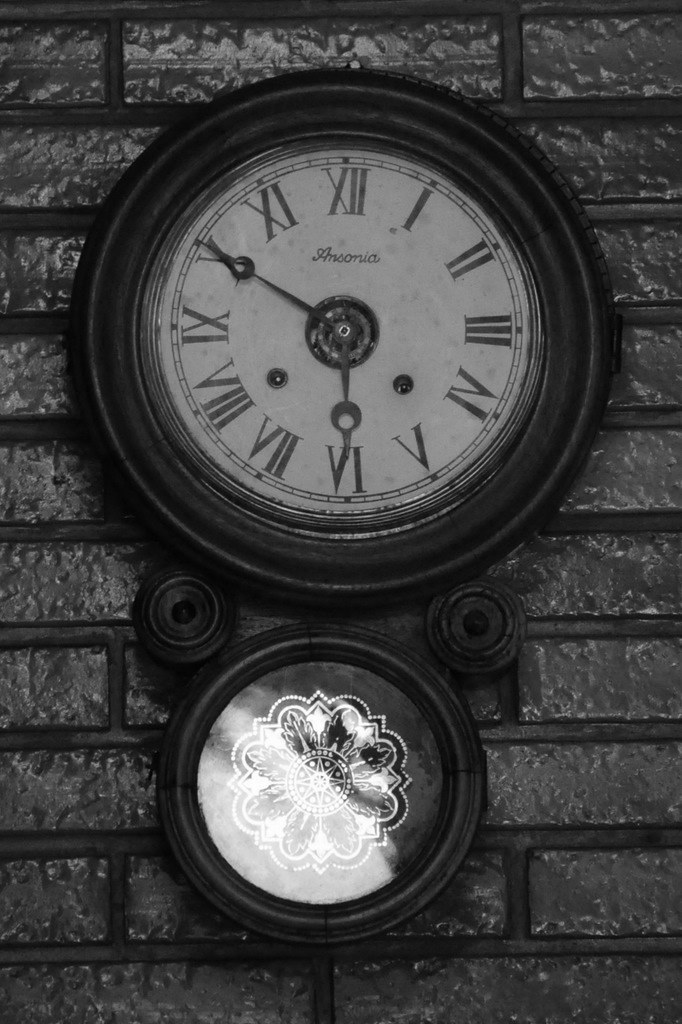The image depicts a black and white photograph of a circular clock mounted on a black, freshly painted brick wall. The clock, positioned about an inch from the top of the frame, features a bold black border and a white clock face adorned with black Roman numerals—I, II, III, IV, V, VI, VII, VIII, IX. The hands of the clock point to 6:50. The clock's center allows a glimpse into its inner workings, with additional small openings visible down left and down right of the clock's face. Beneath the clock, two black circles flank either side, each extending downwards to a smaller black-bordered circle with a glass front. This smaller circle showcases an intricate flower design rendered in black and silver. Overall, the image captures an impressive and detailed timepiece set against a striking, monochromatic backdrop.